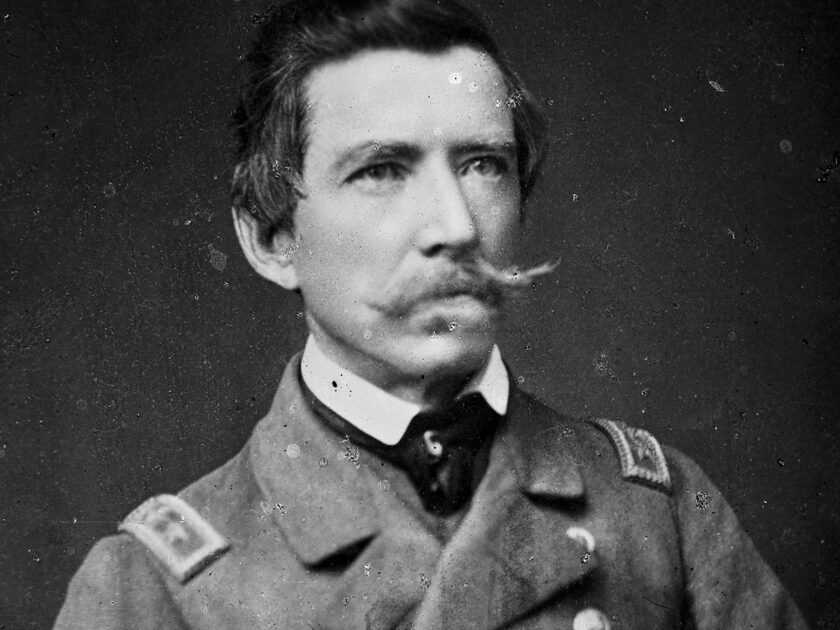This detailed black and white vintage photograph features Rear Admiral Raphael Sims of the Navy. The landscape-oriented image, which appears to be an old and scanned portrait, is speckled and marked with water spots and smudges from aging and development. The man is centrally positioned, looking up and to the right. His dark hair, combed up and back, partially covers the ears and thickens around the temples. He has a handlebar mustache and dark, sunken eyes beneath thick eyebrows. He is dressed in a distinguished military uniform comprising a double-breasted coat with large round brass buttons, shoulder decorations, and a black ascot scarf tied around his neck over a stand-up white collar. This closely framed photograph shows him from the top of his head to just below his shoulders, emphasizing the detailed textures and elements of his attire and facial features.